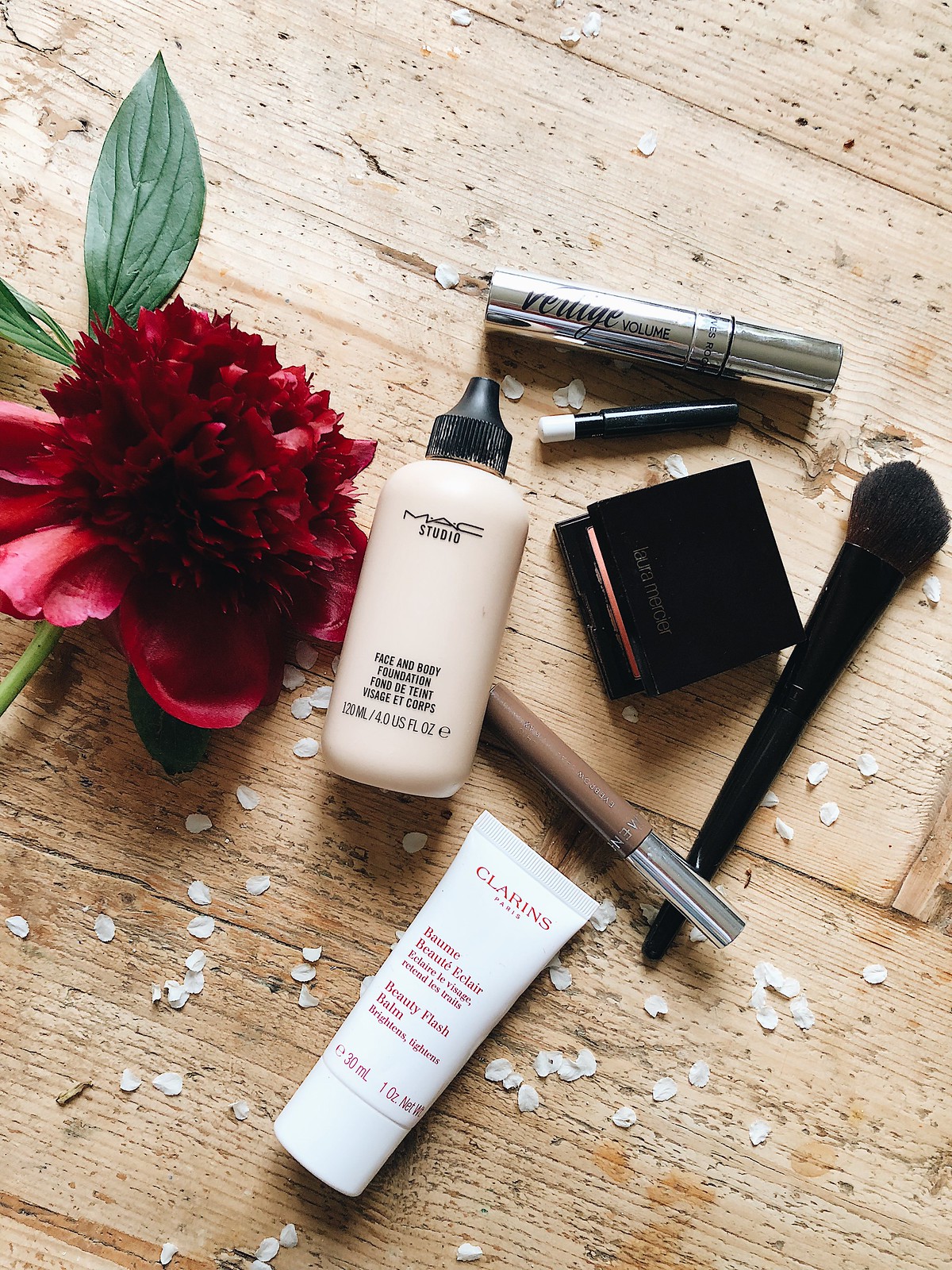The color photograph displays a well-arranged yet seemingly casual assortment of makeup items and a flower on a light-colored wooden surface. The flower, a striking dark red bloom with lush green leaves and a stem, is laid diagonally across the center of the image, extending off the left-hand side. Surrounding the flower on the right are various makeup products: a MAC Studio foundation, a compact from Laura Mercier, a Clarins beauty balm, a mascara, a brown lip gloss, an unidentified black cylinder with a white tip, and a black blush brush likely intended for the compact. Scattered amongst the makeup are small white flower petals, adding a delicate, whimsical touch to the composition. The overall setting exudes an artistic blend of natural beauty and cosmetic elegance.